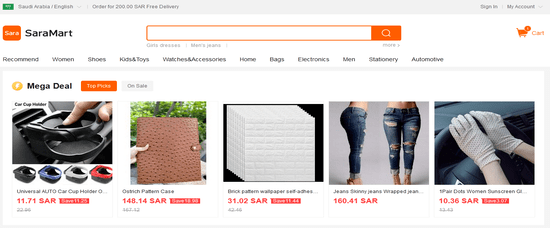Here is a refined and detailed caption for the described image:

---

The image appears to be a slightly blurry screenshot taken from a website with a predominantly white backdrop. In the top left corner, there is a green-colored bar with white text inside it, accompanied by black writing adjacent to it. This section likely includes an address and the phrase "Free Delivery." Following a space, on the right-hand side of the page, "Sign In" and "My Account" with a dropdown arrow are written in black.

Beneath this header, an orange box with white text spells "S-A-R-A," followed by the black text "Sarah Mart." Next to this, there is an orange search bar, accompanied by an orange box with a white magnifying glass icon inside it. To the right of the search bar, a cart icon labelled "Cart" in orange is displayed.

Below this, a black horizontal menu features several categories: "Recommended," "Women," "Shoes," "Kids & Toys," "Watches & Accessories," "Home," "Bags," "Electronics," "Men," "Stationery," and "Automotive." Underneath the menu, a text reads "Mega Deals" in black with an adjacent orange box featuring white writing. Beside this, a gray box labeled "On Sale" in black text is also present.

A row of product pictures follows, starting with:

1. A car cup holder priced at 11.71 SAR.
2. A brown leather-bound journal secured with a clasp, priced at 148.14 SAR.
3. A white rectangular object priced at 31.02 SAR.
4. A woman wearing ripped jeans, priced at 160.XX SAR.
5. A pair of white gloves gripping a car steering wheel.

Each product image is accompanied by its respective price in SAR (Saudi Arabian Riyal).

---